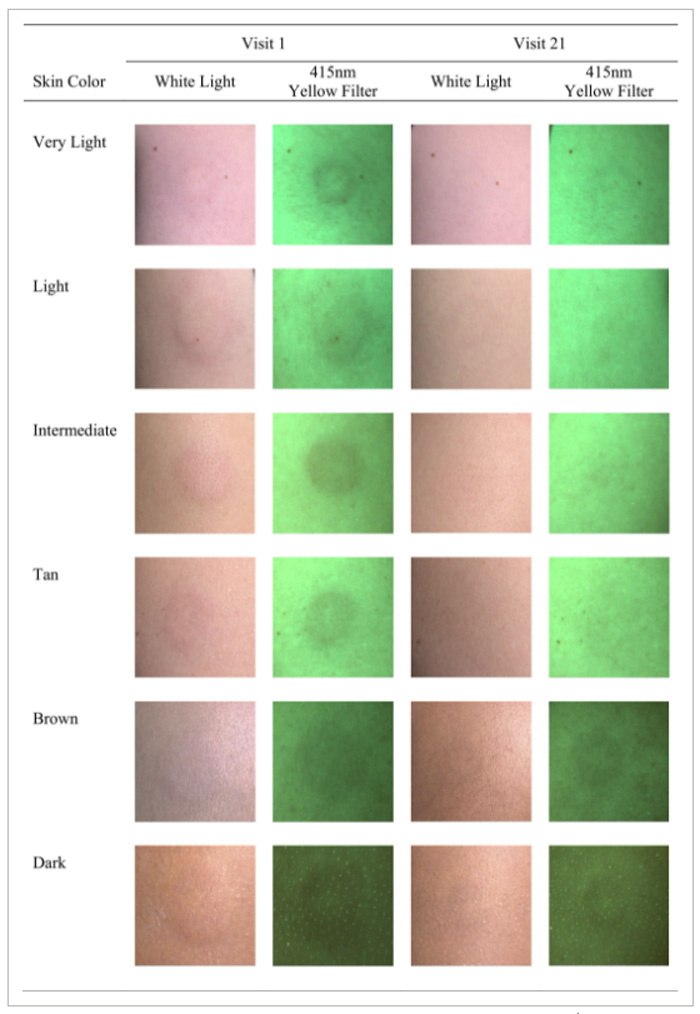The detailed image displays a scientific, medical comparison of skin conditions over time, specifically captured across different visits using specialized photographic techniques. The background is plain white and bordered by a black line, framing a tall rectangular layout. Across the top, labels read "Visit 1" and "Visit 21," signifying two different time points. The left side of the image lists a range of skin tones: very light, light, intermediate, tan, brown, and dark.

The image is divided into multiple rows and columns, likely four by six, with each cell representing a small patch of skin, potentially showing variations such as a rash or bump, which might be indicative of conditions like bruises or ringworm. The first column under visit 1 shows unfiltered skin patches. The second column is under a yellow filter at 415 NM, followed by the third column with white light, and then another 415 NM yellow filter column. The same pattern repeats for visit 21.

The bruises or rashes depicted in the images appear to change over time, diminishing significantly by visit 21. Each photograph was precisely captured using a Canon T6i SLR camera with a 50mm fixed lens set to f/2.2, ISO 400, and variable shutter speed, accompanied by a yellow filter to enhance visibility of the skin changes. The progression from showing clear signs of skin conditions in the initial visit to barely noticeable marks in the final visit illustrates the healing process effectively.